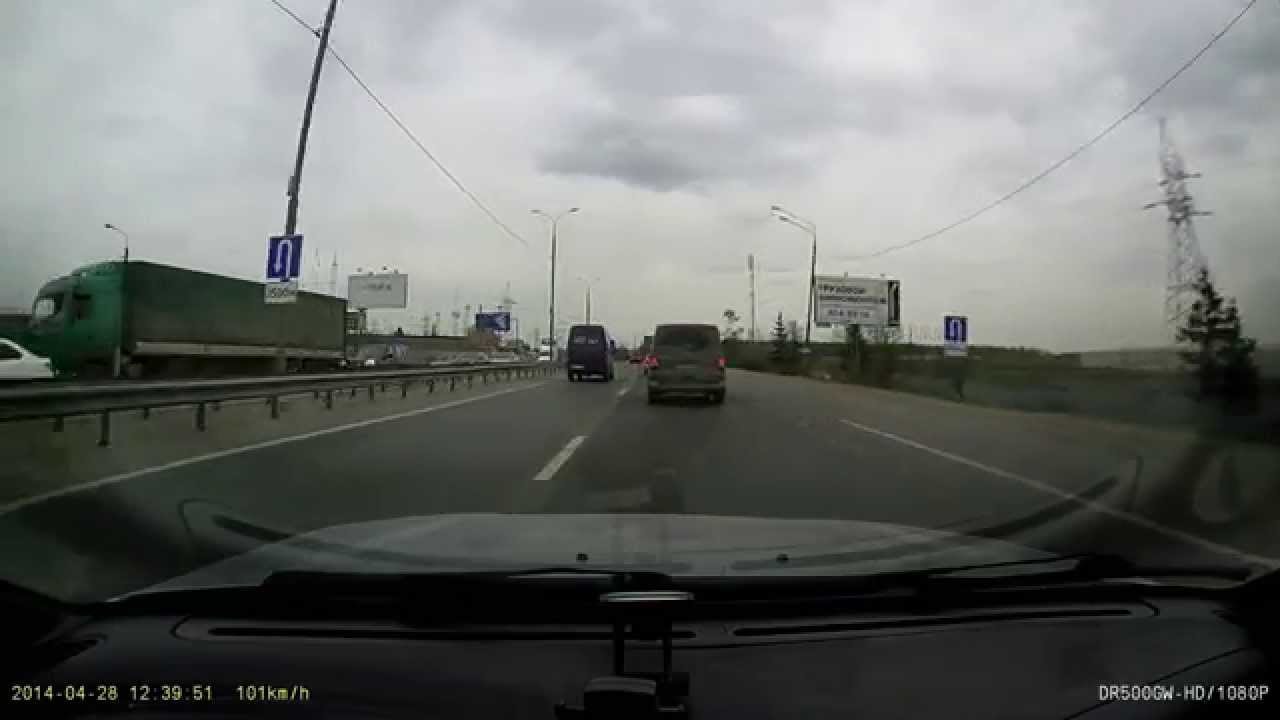The photograph captures a scene from the inside of a vehicle, as indicated by the timestamp "12:39:51" on April 28, 2014. The sky is overcast, casting a grayish hue over the daytime landscape. The vehicle's windows appear to be tinted, providing a shaded view of the outside world. Traffic moves in both directions on the road, with a couple of vehicles visible ahead in the same lane, while a green truck and a white car are traveling in the opposite direction.

Billboards line the sides of the road, offering a glimpse into the commercial activity of the area. Additional signage indicating U-turns can be seen both close by and further down the road. In the distance, a cell phone tower is faintly visible on the right-hand side. Power lines stretch along each side of the road, while street lamps dot both sides of the highway, highlighting the infrastructural elements that accompany the traffic scene.